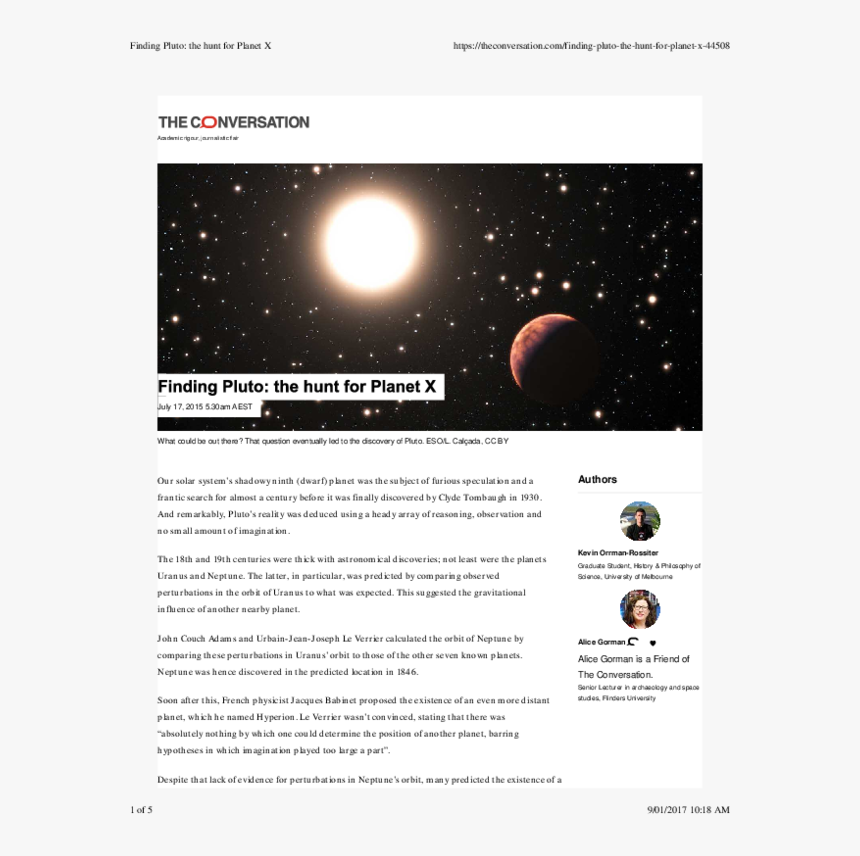In this captivating image, we see an article titled "Finding Pluto: The Hunt for Planet X" prominently displayed. The top left corner features the bold title "Finding Pluto: The Hunt for Planet X," while on the right side, the URL "theconversation.com" is clearly visible, indicating the source of the article.

The centerpiece of the article is an enthralling image of a galaxy adorned with several planets, encapsulating the cosmic theme. Below this striking image is the captivating subtitle: "What could be out there? The question eventually led to the discovery of Pluto."

The body of the article delves into the historic pursuit of Pluto, a solar system's shadow dwarf planet that intrigued astronomers and sparked fervent speculation for almost a century. The relentless search culminated with its discovery by Clyde Tombaugh in 1930. Remarkably, this discovery was achieved through a combination of reasoning, observation, and a considerable amount of imagination.

The narrative recounts the rich history of astronomical breakthroughs during the 18th and 19th centuries, highlighting the discoveries of Uranus and Neptune. Notably, Neptune's existence was predicted through observed perturbations in Uranus's orbit, attributed to the gravitational influence of a neighboring planet. Astronomers John Couch Adams and Joseph Le Verrier calculated Neptune's orbit based on these perturbations, leading to its discovery in the predicted location in 1846.

The article also mentions French physical geographer Jacques Babinet, who proposed the existence of an even more distant planet, which he named Hyperion. 

The authors of this compelling piece, Kevin Ormerod, Rosie, and Alice Gorman, are listed on the right side, accrediting their contributions to this illuminating narrative on the quest for Pluto.